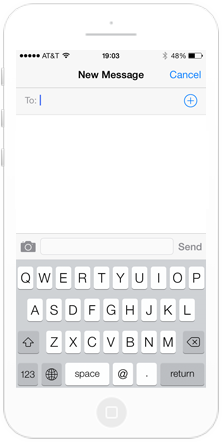This is a detailed image of a smartphone screenshot superimposed onto a cell phone backdrop, both in portrait orientation with rectangular shapes and rounded edges. On the smartphone, three equal-sized buttons are located near the top left, likely for power and volume control. At the screen's top, a gray horizontal bar features five circular icons, the carrier name "AT&T," and a fully filled Wi-Fi meter. In the middle of this bar, the time reads "19:03," accompanied by a Bluetooth icon, "48%" in text, and a horizontal battery icon indicating 48% charge.

Below this bar, a black header reads "New Message" with a blue "Cancel" button on the right. A gray horizontal line separates this header from the main interface, which starts with a field labeled "2" on the left, a blue scroll cursor, and a drop-down menu.

The central part of the screen displays a blank white space, presumably for composing a message, followed by a keyboard popup. This keyboard includes a camera icon to the left, a central white search bar, and a gray "Send" button. The QWERTY keyboard features white keys, black letters, and a gray background, with a "Return" button and various useful symbols at the bottom.